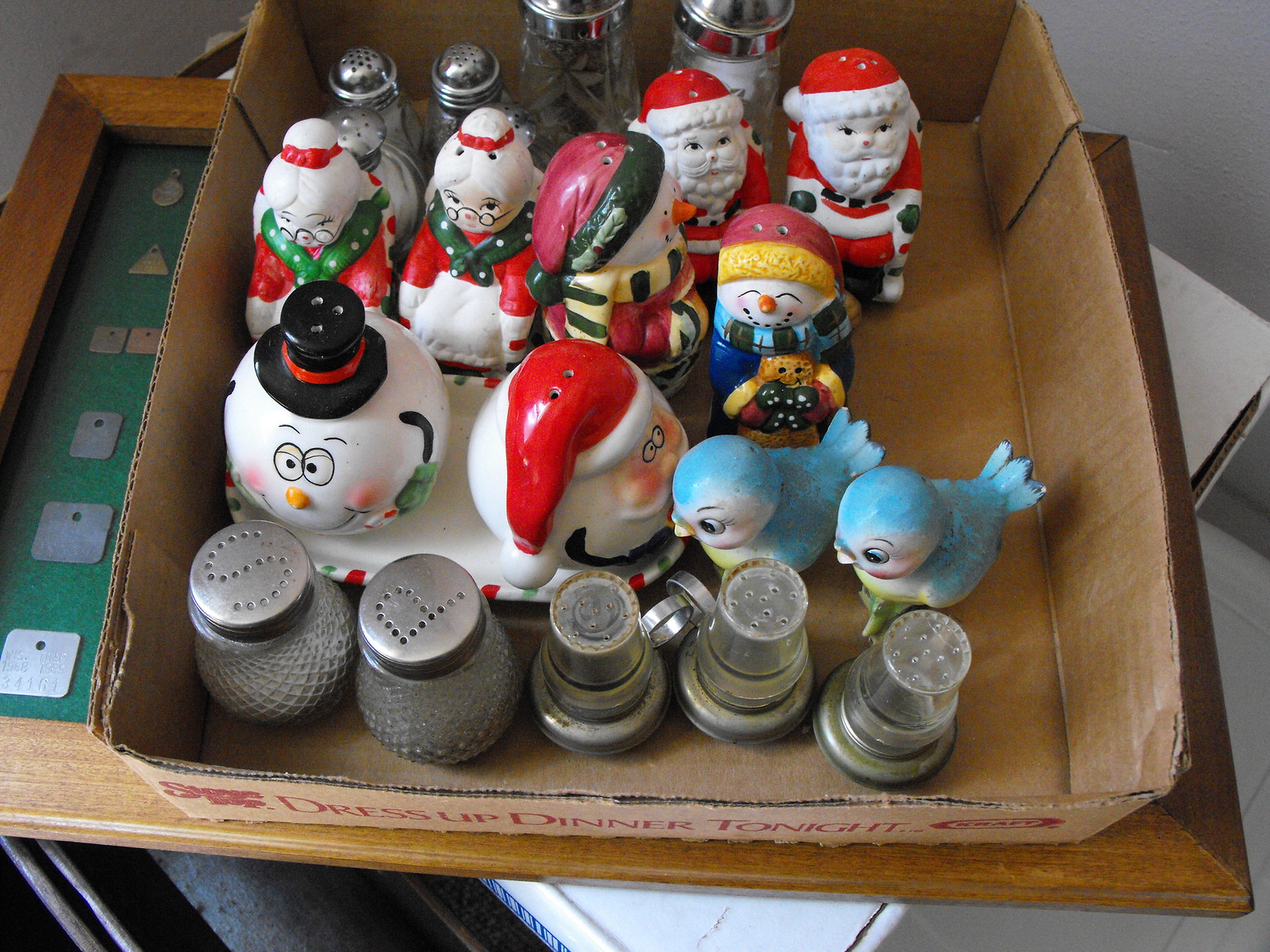Inside a shallow, repurposed brown cardboard box labeled "Craft Dress Up Dinner Tonight," there is a diverse collection of salt and pepper shakers. The box, typically used for storing drinks, now holds an array of both traditional and novelty shakers. In the front row, there are classic glass shakers with silver lids labeled "S" and "P." Behind these, a variety of Christmas-themed salt and pepper shakers are displayed, including two sets featuring the full bodies of Santa Claus and Mrs. Claus, as well as several snowmen decked out in red hats, scarves, and sweaters. There are also unique shakers shaped like bluebirds, along with more distinctive pieces featuring just the heads of Santa and a snowman in a cartoony style. Below the box, a wooden picture frame with a green insert and partially obscured metallic tags can be seen.